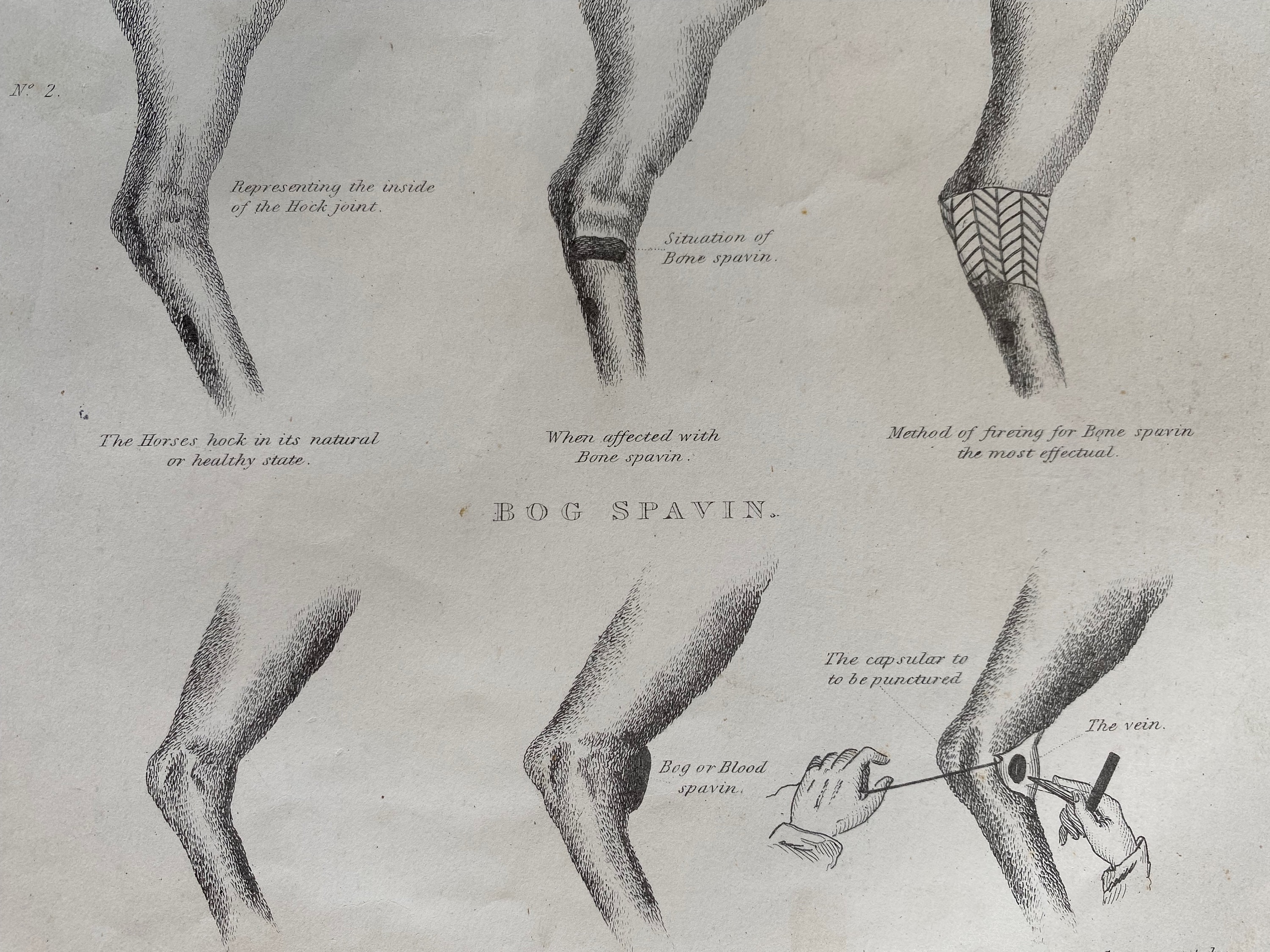The image is a page from an older book about animal medicine, specifically focusing on the treatment of a horse's hock joint. The detailed black-and-white diagrams are arranged in two rows of three, with the upper left diagram labeled with the number two. Each drawing portrays different conditions and treatment methods for the hock joint.

The top left diagram illustrates the horse's hock in its natural or healthy state, labeled "the horse's hock in its natural or healthy state." Adjacent to it, the upper middle diagram shows a cutaway view of the joint, labeled "representing the inside of the joint," while the upper right diagram details "method of firing for bone spavin, the most effectual,” illustrating a significant portion of the leg.

On the bottom row, the diagrams from left to right depict the progression of a condition called bone spavin, with captions like “situation of bone spavin” and “when affected with bone spavin.” The bottom middle shows a condition described as "bog spavin," a large growth on the leg. The bottom right diagram illustrates a technique involving suturing or puncturing, where human hands are depicted working with a needle and thread on the affected area.

Illegible black cursive writing accompanies each diagram, adding further notes or details. Overall, this intricately detailed illustration provides a comprehensive look at various states and treatments of the horse's hock joint.